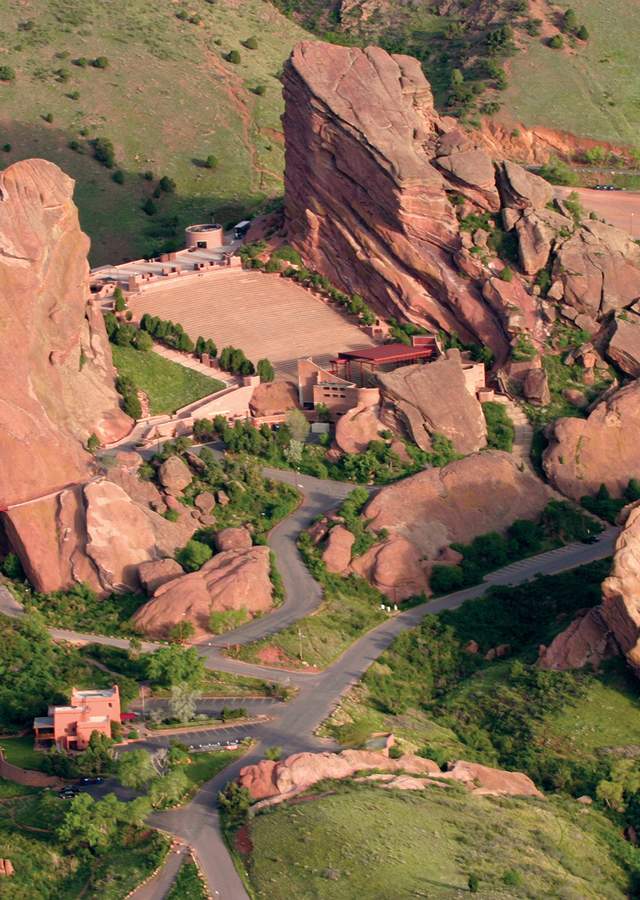The photograph captures a sprawling amphitheater nestled amidst striking natural rock formations. The perspective looks down on a verdant area with vibrant green grass that contrasts sharply with the rugged terrain. Prominently, two towering, pinkish rock formations frame the scene on either side, creating a dramatic backdrop. Near the lower left corner, a red brick or adobe building with a flat roof stands out. 

A series of roads extend through the area, with one leading directly to the amphitheater. The stage of the amphitheater, which is closer to the camera, has a reddish roof. Surrounding the stage, the steps of the seating area are a light pink color, harmonizing with the natural rock hues. A cylindrical building is visible atop the rock formations, accessible by a stairway to the right of the stage. 

The area is enveloped in lush greenery, with patches of green shrubs adding to the natural beauty. Beyond the immediate amphitheater complex, a gray cement road stretches into the distance, flanked by the imposing rock formations. The distant landscape features more reddish-brown rocks and a clearing of light rock, enhancing the rugged and picturesque scenery.